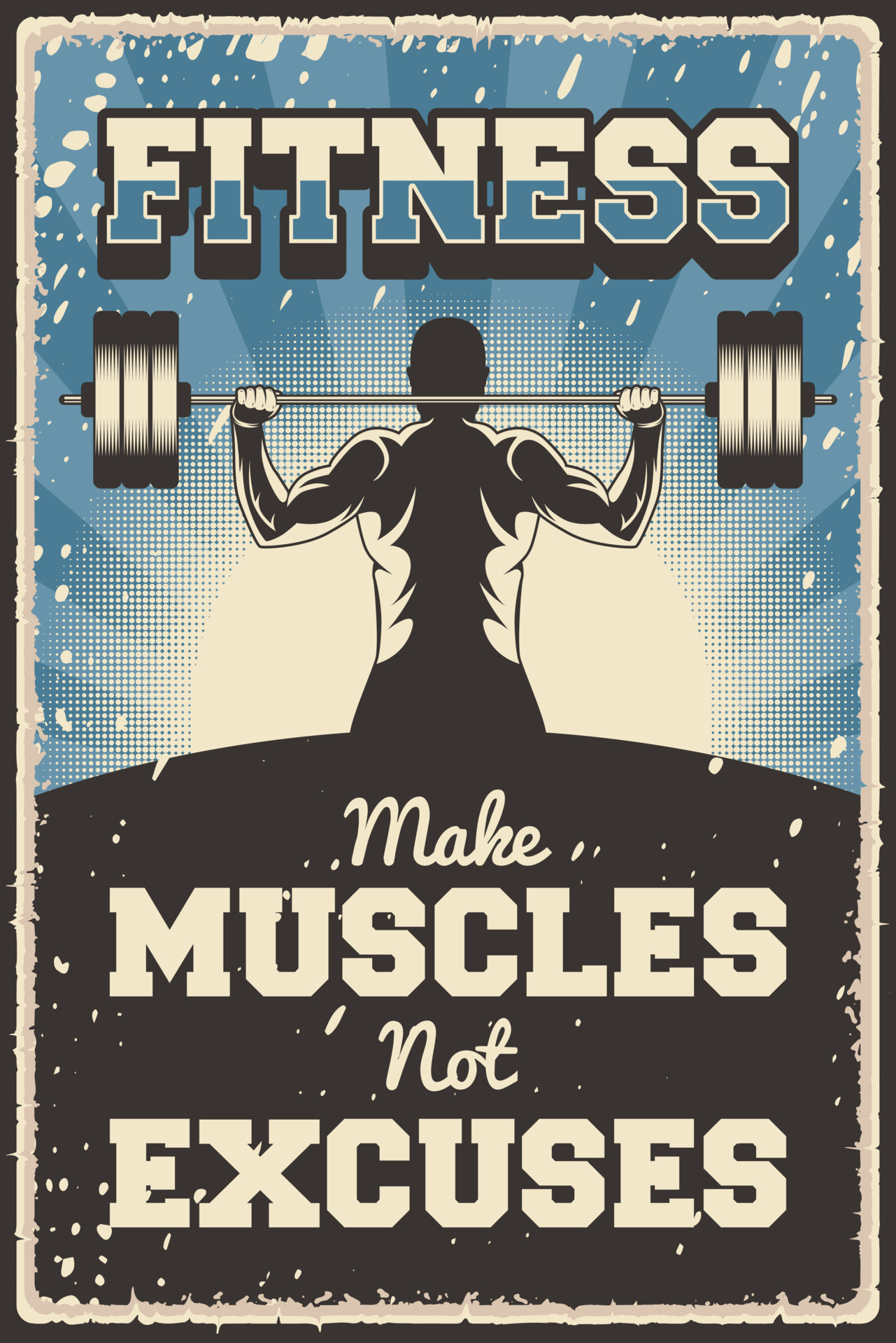The fitness poster features a black outer border and a white inner border, with a predominantly blue and black color scheme. The top of the poster showcases a radiating light blue background with beige speckles. At the top, "Fitness" is prominently displayed in large, multicolored letters that fade from light tan to blue, set against a black background. Below this text, an image of a muscular weightlifter is depicted from behind. The man is holding a barbell loaded with three weights on each side, positioned at neck height, highlighting his well-defined muscles. At the bottom of the poster, against a black backdrop, the motivational phrase "Make muscles, not excuses" is written in large white font. The overall design is professional and impactful, aiming to inspire and motivate viewers.